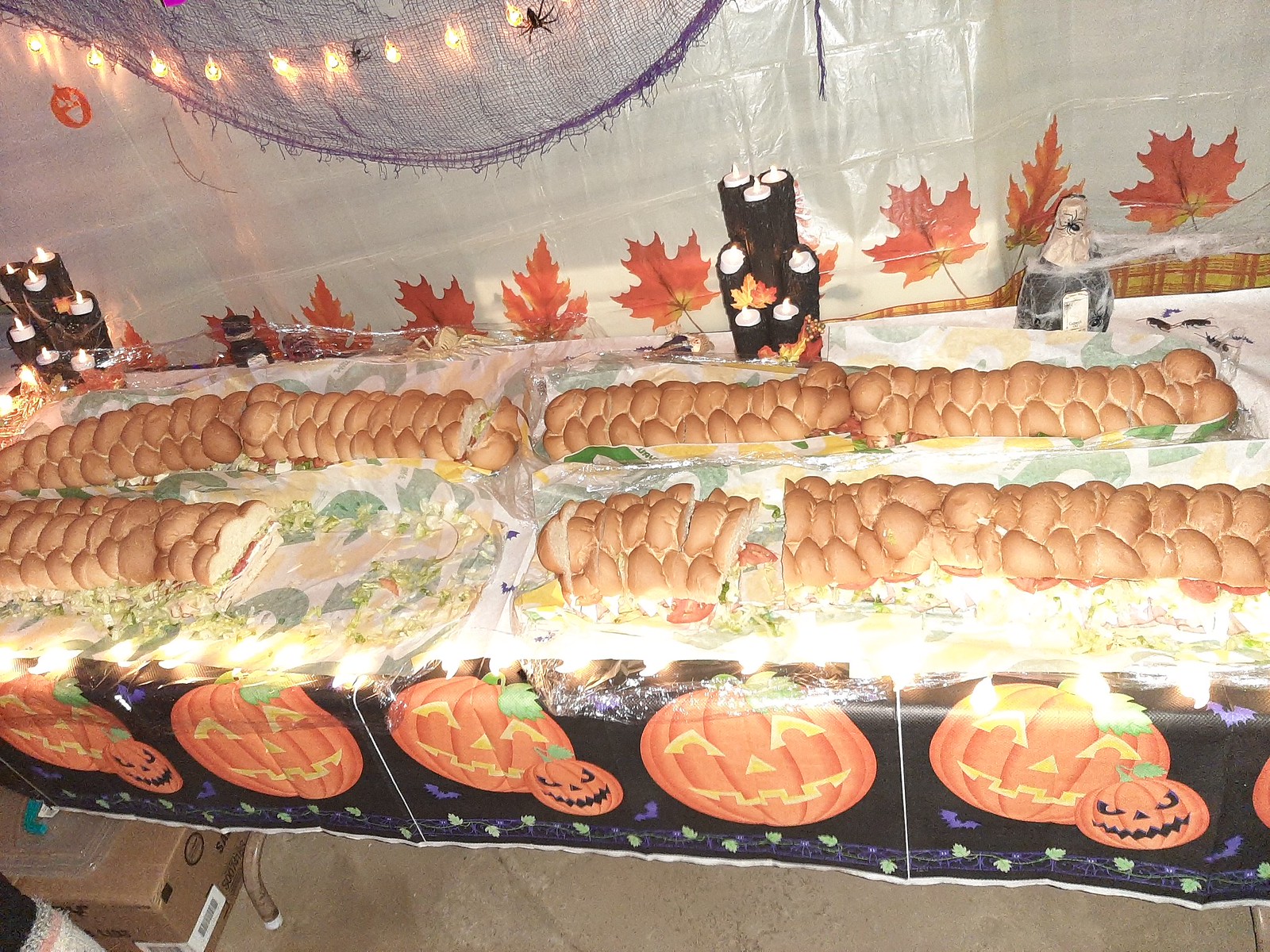The image depicts a festive Halloween-themed banquet table adorned with a variety of decor and food. The focal point is a spread of sub sandwiches made with challah bread, featuring visible layers of lettuce, tomatoes, and meat. The sandwiches are arranged on a plastic tablecloth that transitions from a light color on top to a black background with orange pumpkins and intricate jack-o'-lantern designs. The table itself appears to be long, possibly made up of multiple tables or a lengthy bench-type table.

Above the table, string lights with tiny spiders drape across, adding a spooky ambiance. At the far end, there are black candle holders with white LED candles grouped together, adding a touch of eerie light without an actual flame. The background is decorated with a fall leaf wall hanging of orange and yellow maple and oak leaves, giving a seasonal feel. Purple netting with fake spiders and an intricately woven blue spider web complete the backdrop, alongside a cardboard box peeking out from underneath the table. The Halloween tablecloth also features small fake bugs, enhancing the creepy festivity of the setup.